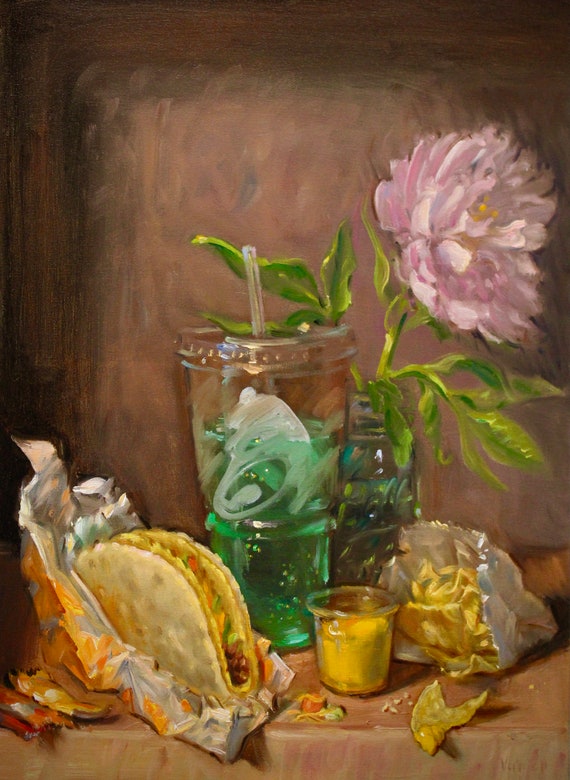A very detailed and amusing painting, resembling an elegant, old-fashioned still life, captures a Taco Bell meal against a brown, rustic background. In the scene, there is a clear glass jar branded "Ball" containing a delicate pink flower with yellow accents and green leaves, presenting a charming contrast to the fast food items. To the right, a disposable plastic Taco Bell cup, adorned with the recognizable emblem, holds a teal-green liquid, possibly Mountain Dew, complete with a straw. The main food focus is a Gordita Crunch, a hard taco shell wrapped in a soft one, partially unwrapped to reveal a colorful mix of red fillings, yellow cheese, and green lettuce. This is complemented by three Taco Bell sauce packets in red, orange, and yellow, alongside a small container of nacho cheese and a white paper bag filled with tortilla chips. The overall composition playfully merges the elegance of classical still life with the modern, everyday appeal of fast food.